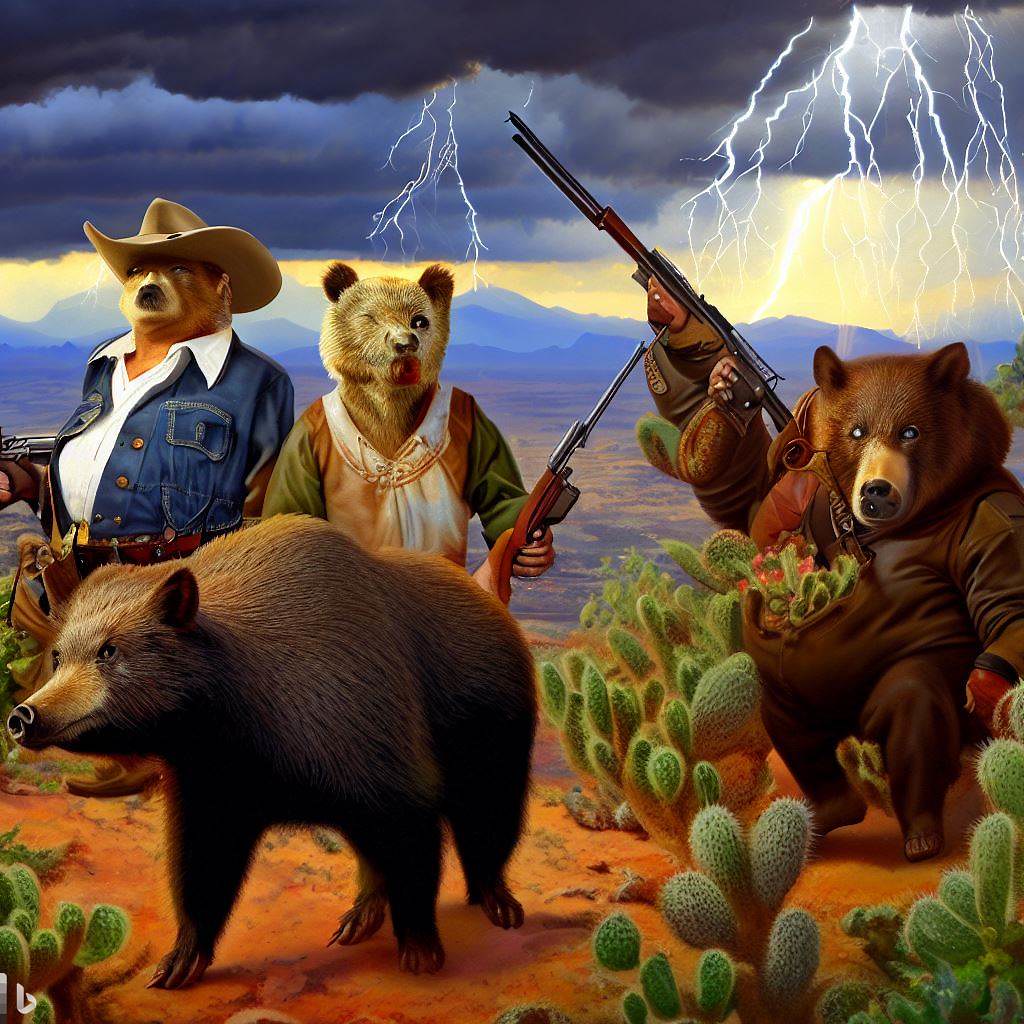This is a highly detailed and animated scene reminiscent of an Old West setting, featuring anthropomorphic bears. In a desert landscape with reddish-orange soil, scattered cacti, and distant purple mountains, four distinct bears are depicted under a dramatic sky filled with dark, brooding clouds and sharp bolts of white lightning.

In the foreground, a dark brown bear on all fours, with a tan snout and an unusual nose, contrasts the human-like postures of the bears behind it. This wild bear is one of the few elements not dressed in clothing.

To the back left, a bear dressed as a cowboy stands upright. He wears a white shirt, a denim jean jacket, and a cowboy hat, complete with a gun belt and a weapon in hand. This bear, resembling a sheriff, oversees the scene with authority.

Next to him, a female bear is dressed in a white smock with green sleeves, one eye closed as if winking or injured. She holds a rifle, and a red object protrudes from her mouth, adding a touch of mystery and grit.

Further to the right, a hefty brown bear wears a brown jumpsuit. This bear, also armed with a rifle pointed skyward, adds to the scene's tension, gazing directly at the viewer.

The background features dramatic weather elements, including jagged lightning bolts striking from dark clouds overhead, casting an ominous tone over the colorful yet desolate desert terrain. This blend of rugged natural beauty and the anthropomorphized characters creates an intriguing and whimsical artwork full of narrative potential.